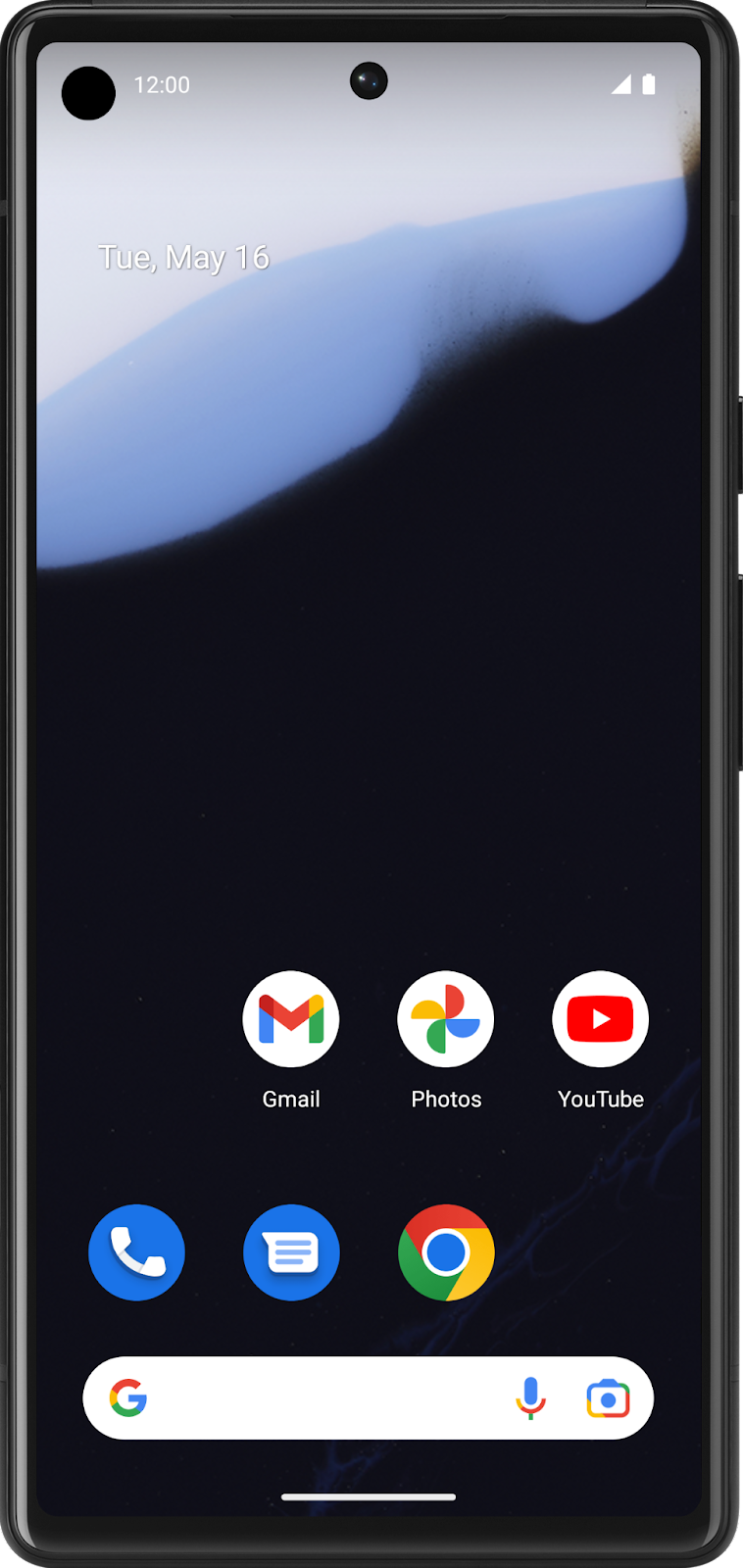This detailed caption describes an image of a black cell phone:

"This image features a sleek black cell phone. At the top left corner of the screen, there is a small black circle indicating the time, which is set to 12 o'clock. Also at the top, but centrally located, is another black circle that likely contains the front-facing camera. On the top right corner, a full battery icon is displayed. The phone's screensaver transitions from the bottom to the top, starting with black hills, merging into a blue gradient, and finally turning light gray. On the light gray background near the top, the date is displayed in white text: 'TUE, MAY 16'. 

At the bottom part of the screen, a row of frequently used apps is visible, including Gmail, Photos, and YouTube. Below these apps, there are three circular icons: a blue circle with a phone symbol, a blue circle with a chat mobile icon, and a colorful circle representing the Google app. Underneath this row, there is a white section designated for the Google search bar, followed by a thin white line marking the bottom edge of the display."